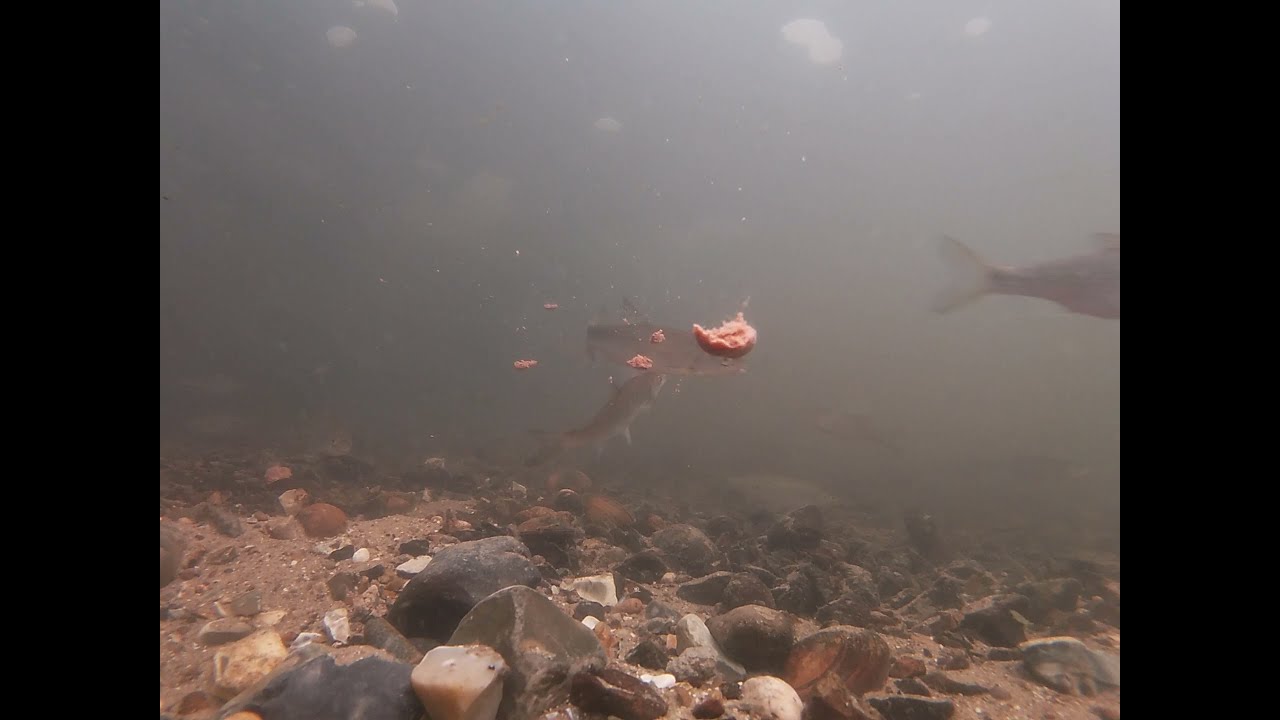In this underwater photograph, the top two-thirds of the image are dominated by a hazy, bluish-gray water that's slightly murky and dirty. Within this water, globs of pinkish raw meat float, seemingly attracting several fish. In particular, three fish are distinguishable: one fish swims near the center while another lurks somewhat further beyond the meat, and the back half of a larger fish with visible tail fins can be seen in the left-hand corner of the image. The bottom of this underwater scene features a diverse array of rocks in various colors including white, gray, black, and orange, interspersed with sand and debris, giving the base a very rugged and natural appearance. The overall image is somewhat fuzzy, giving a sense of depth and mystery to the underwater environment.